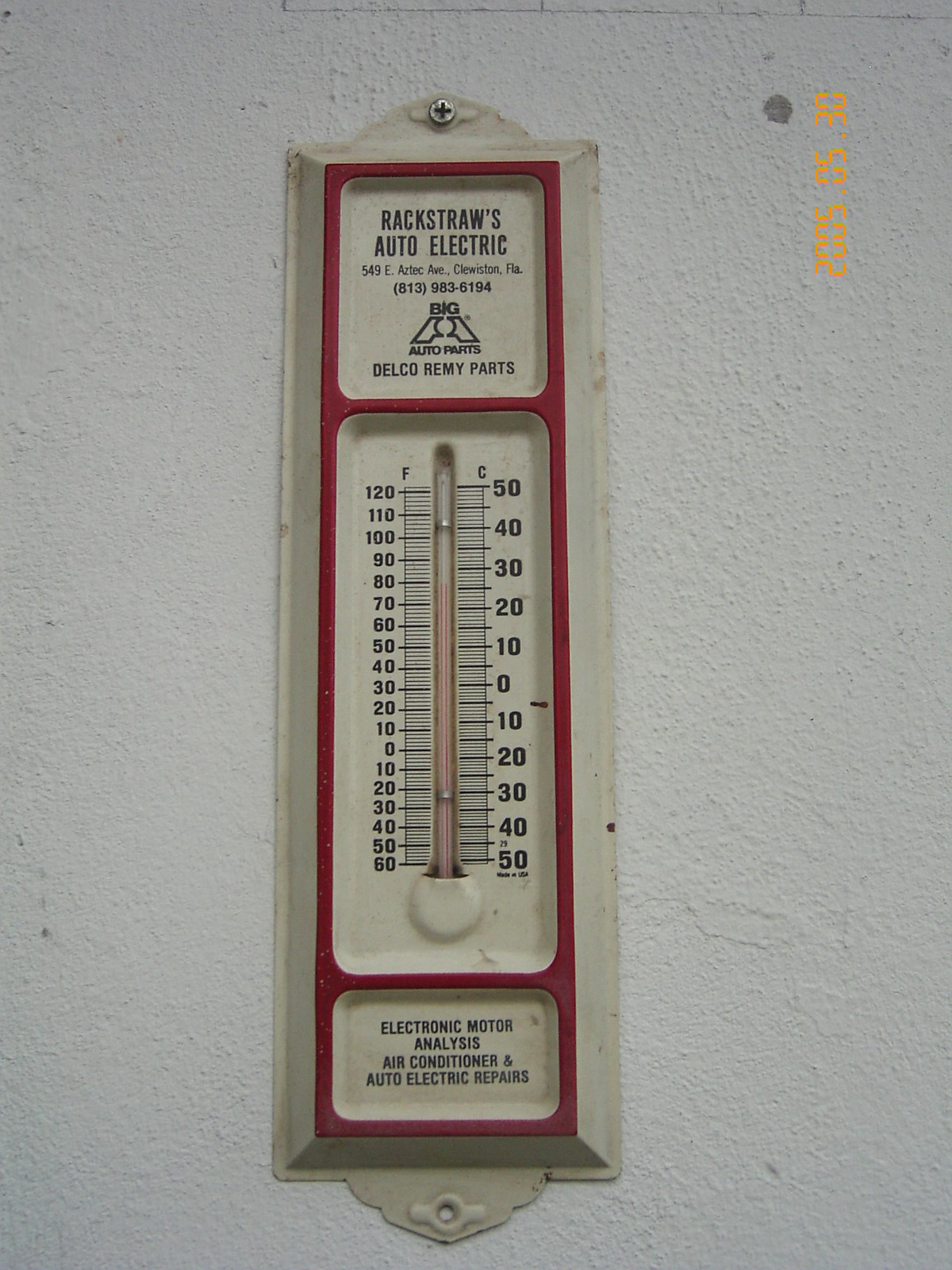A photograph captures an outdoor thermometer affixed to a white, textured plaster wall. The thermometer is crafted from white metal and features a long, rectangular design divided into three distinct segments bordered in red. At the top segment, the inscription "Rackstraws Auto Electric" is prominently displayed in black letters, followed by the address and phone number. Below that, it reads "Big Auto Parts" and includes a symbol with "Delco Remy Parts." The central section houses the thermometer itself, marked with Fahrenheit degrees on the left and Celsius degrees on the right, showing a current temperature of approximately 78°F. The bottom segment advertises "Electronic Motor Analysis, Air Conditioner, and Auto Electric Repairs." Additionally, an orange timestamp is visible in the top right corner of the image.